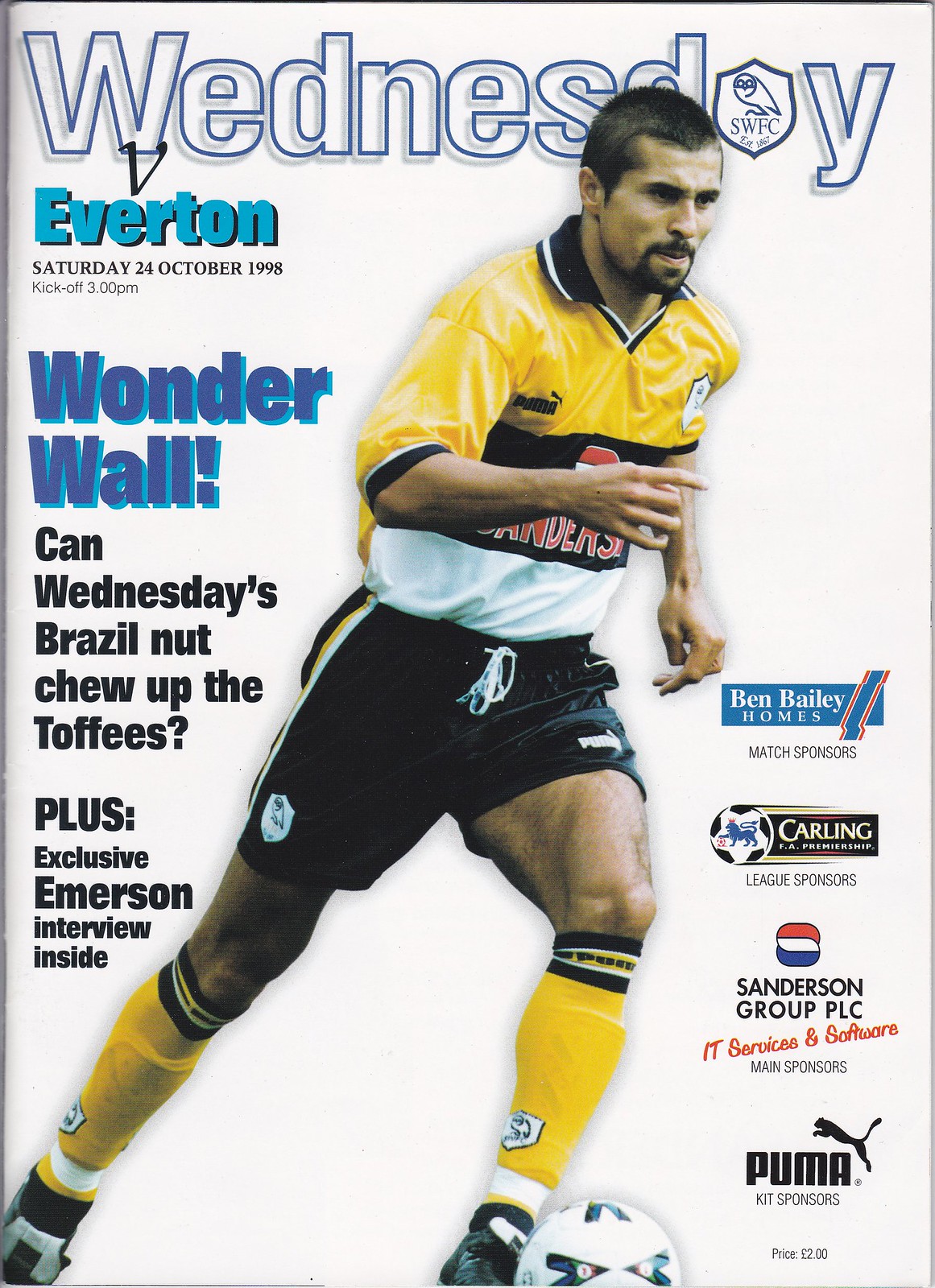The cover of the magazine features a vibrant color-printed photograph of a male soccer player, likely Hispanic, donning a modern yellow, black, and white striped jersey, black shorts, and yellow socks. The player, with brown hair and a black mustache and beard, is captured mid-action, running towards the right and kicking a soccer ball, partly cut off at the bottom of the image. The dynamic background has a slight pinkish tint, adding to the energetic feel of the cover.

Prominently displayed at the top is the headline "Wednesday," styled in white with a blue outline and a gray drop shadow. Beneath that, the word "Everton" appears in bright blue with a black shadow, followed by the date and kickoff time: "Saturday, 24th October 1998, 3 p.m." In bold dark blue text, the headline "Wonderwall" stands out, with a quirky subheading in black text asking, "Can Wednesday's Brazil nut chew up the toffees?" Further down, another subheading reads, "Plus exclusive Emerson interview inside." The background of the text is blue and black with some white and a touch of red. The lower right corner of the cover features four sponsor logos and a price tag of two pounds.